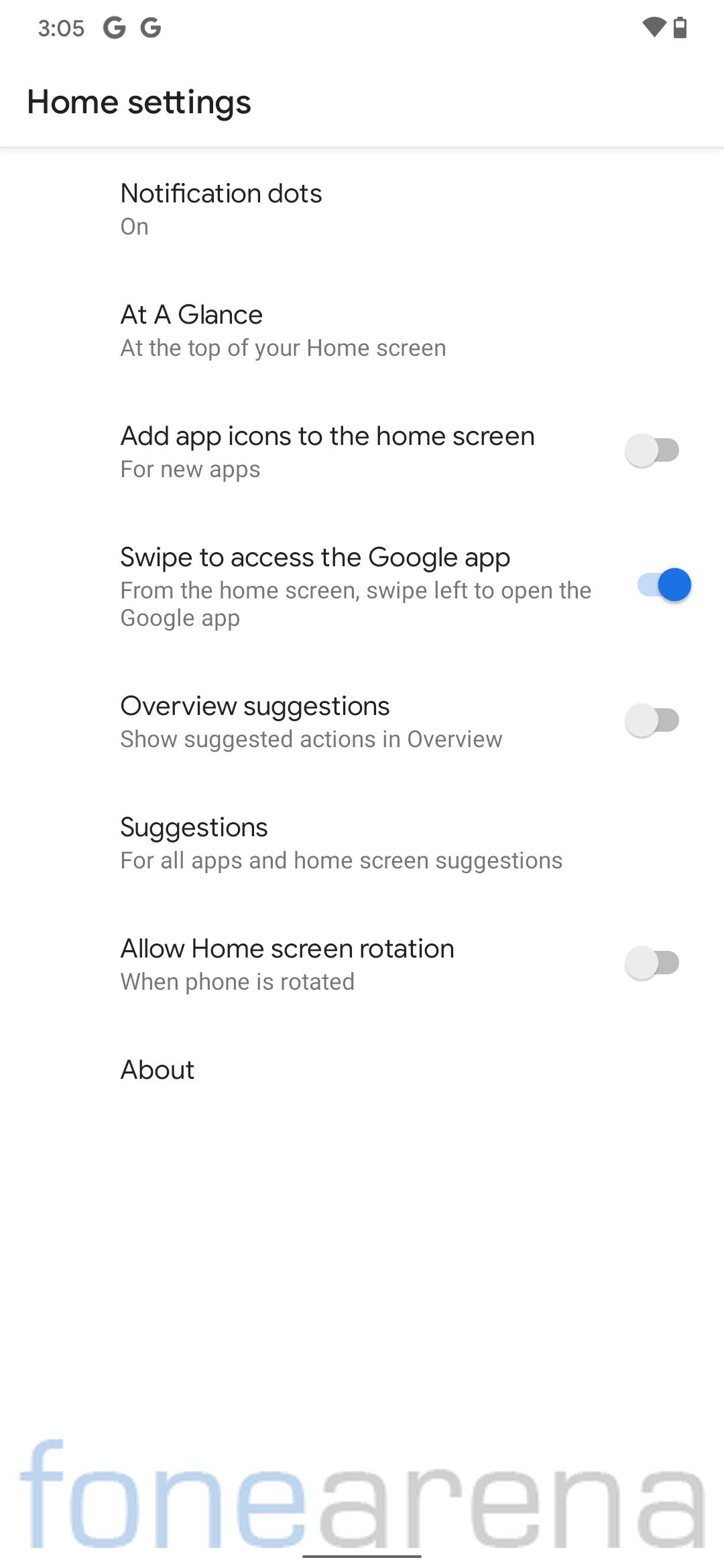This screenshot displays a cell phone interface, captured at 3:05 PM. In the upper left corner, the time "3:05" is clearly visible. To the right of the time, the Google logo, represented by a "G," appears twice in succession. In the upper right corner, there are icons indicating a strong Wi-Fi connection and a nearly full battery.

Directly below these icons, the word "Home" appears in black font with a capital "H," followed by a gray separator bar. This leads to the first option labeled "Notification Dots," which shows as "On." 

Below, the "At a Glance" feature states that it is displayed at the top of the home screen. The option to "Add App Icons to the home screen" is currently toggled off. Furthermore, the "Swipe to access the Google app" feature is active, while the "Overview Suggestions" option is turned off. 

Overall, the screenshot provides a detailed look at various settings and visual indicators on the phone's interface.